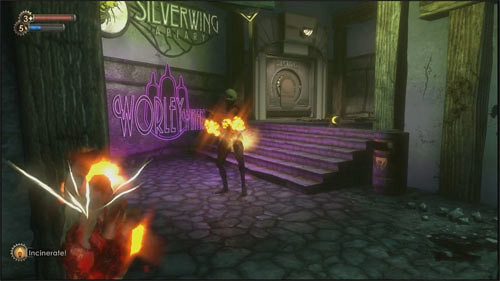In this rectangular image, which appears to be a snapshot or screenshot from a video game, two characters are prominently featured. The character in the foreground is facing the camera, standing confidently with flames encircling their wrists or hands. The second character, positioned in the bottom right with their back to the camera, is illuminated in various vibrant colors, though their head is not visible. The background showcases a detailed wall with neon signage, including "Silver Wing Apparel" in a greenish-yellow hue and "Whirly" in a striking purple. Purple steps ascend in the middle of the scene, possibly leading to a door or entrance above, contributing to the intriguing environment.